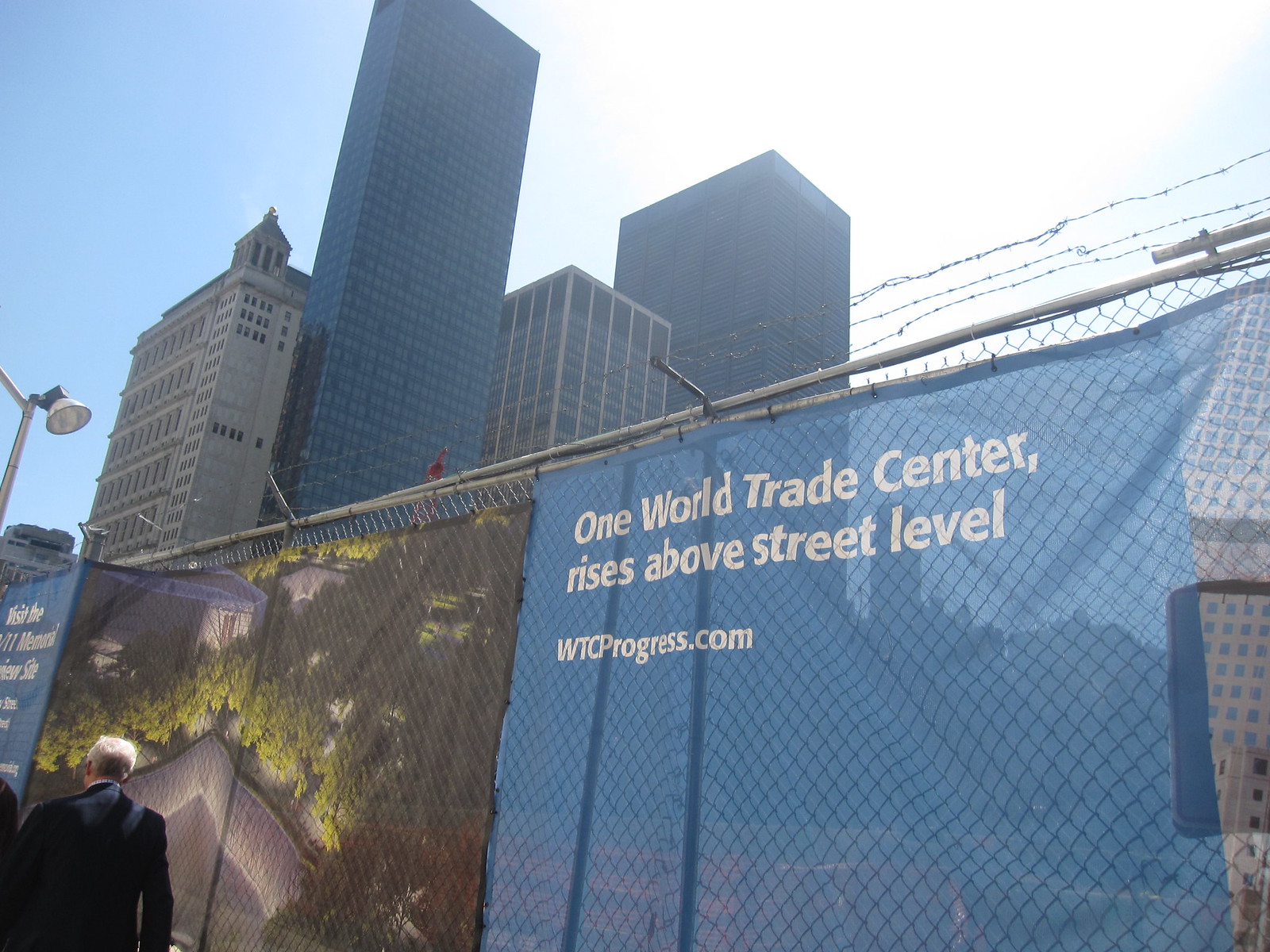This photograph captures a sunny blue sky day with several high-rise buildings extending vertically from the left and center of the image. In the foreground, there is a chain-link fence topped with barbed wire, which spans horizontally across the frame. On the fence, there are three banners; the first prominent banner is powder blue with white text reading, "One World Trade Center, Rises Above Street Level," followed by the URL "wtcprogress.com". The second banner features a painting depicting houses, trees, and additional structures. The third banner appears to be cut off and is not fully visible. A bird is perched on part of the chain-link fence, adding a touch of life to the industrial scene. Additionally, a street light is positioned on the left side of the photograph. Above the skyline, the sky transitions from a bright blue on the left to a white hue filled with clouds on the right. Notably, one of the high-rise buildings has a distinctive steeple-like top, adding an architectural point of interest.